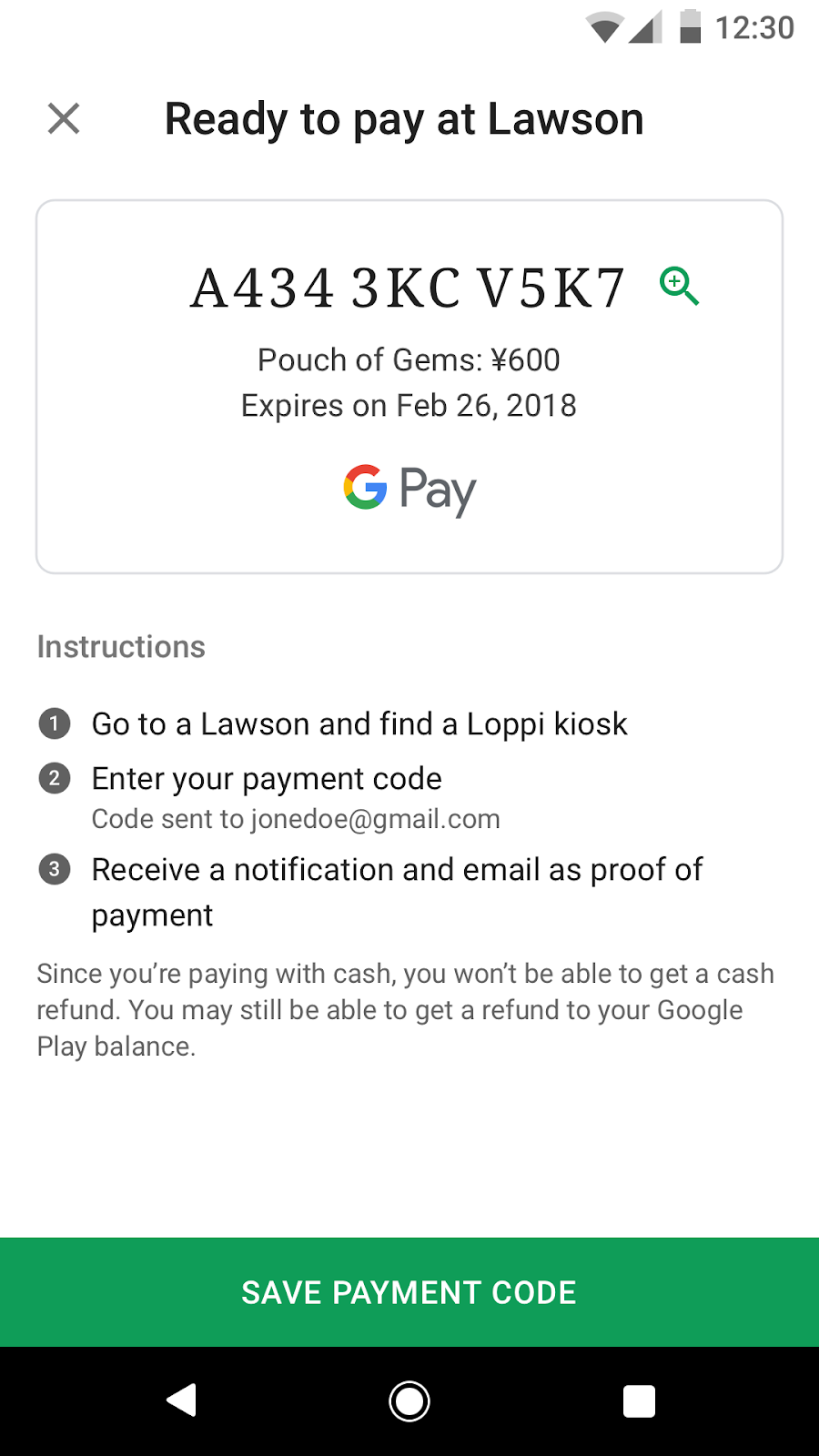The image depicts a smartphone screen showcasing a payment interface for Google Pay. At the top of the screen, typical status indicators for battery life, Wi-Fi signal, and phone signal strength are visible. The time is shown as 12:30.

Beneath the status indicators, there is a notification area labeled, "Ready to pay at Lawson," bordered and organized in a box. Inside this box, a message indicates the user is prepared to make a payment at Lawson using Google Pay. A voucher code is provided, displayed as 'A4343KC' and 'B5K7', along with a magnifying glass icon labeled "Pouch of Gems" followed by a yen symbol (¥) denoting a value of 600. The voucher is noted to expire on February 26, 2018.

Below the payment readiness notification, the interface features a section titled "Instructions." This section provides a step-by-step guide for redeeming the voucher:
1. Go to a Lawson store and locate the LOPPI kiosk.
2. Enter the payment code received via email.
3. Receive a notification email as proof of payment.

A note within the instructions states that since the payment is being made with cash, a cash refund is not possible. However, a refund may still be issued to the user's Google Play account.

At the bottom of the screen, a green button labeled "Save Payment Code" (text in white on a green background) is prominently featured. Below this button are navigation icons: a backspace arrow, a solid circle, and a white square.

Overall, the smartphone screen is displayed on a white background, creating a clean and organized layout that highlights critical information for completing a Google Pay transaction at Lawson.